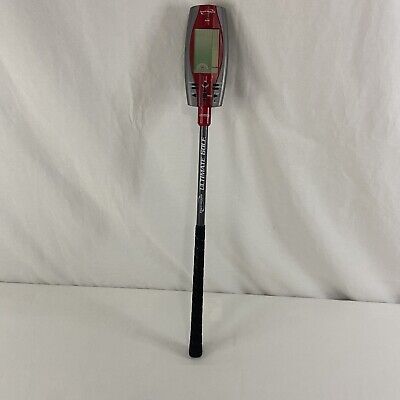This photograph features a unique electronic device, prominently labeled as "Ultimate Pole," leaning against a pristine white backdrop and resting on a matching white floor. The device resembles a long pole, somewhat similar to a cane or a piece of sporting equipment. It extends upward into an electronic box, which houses a maroon and translucent gray LED or LCD display screen, reminiscent of a smaller parking meter. The bottom half of the pole is wrapped in a black, rubberized grip for ease of handling. The setting appears to be indoors, likely under fluorescent lighting, as indicated by the shadows cast by the device. The exact purpose of the device remains unclear, though it could potentially be used for measuring distance or other functions.